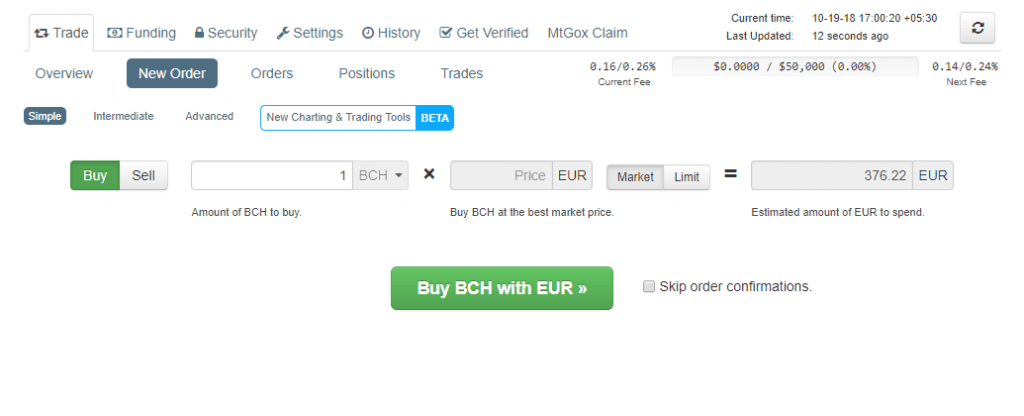A detailed screenshot from a stock trading website or app focused on the "Trade" tab, specifically under the "New Order" subcategory with the "Simple" ordering option selected. The interface is primarily white and includes several navigation tabs at the top: Trade, Funding, Security, Settings, History, Get Verified, and MTGOX Claim. The "New Charting and Trading Tools" button is prominently highlighted with a blue box, indicating its beta status.

In the top right corner, the current time is displayed as October 19, 2018, 17:00:20, with a time zone offset of +05:30. This data is noted to have been last updated 12 seconds ago, and a refresh button is positioned nearby for manual updates. Directly below, the current trading fee is listed as ranging from 0.16% to 0.26%. A box indicating some monetary limits shows a range of $0 to $50,000 at 0% fee. Adjacent to this, the next tier fee is noted as 0.14% to 0.24%.

The main section of the screen features an order form for purchasing Bitcoin Cash (BCH) using Euros (EUR). The "Buy" option is selected, highlighted in green. The order form specifies purchasing 1 BCH at the best market price, translating to an estimated spending amount of 376.22 Euros. At the bottom, a large green button labeled "Buy BCH with Euros" stands out for finalizing the purchase. An unchecked box labeled "skip order confirmations" is also present, giving users the option to streamline their buying process.